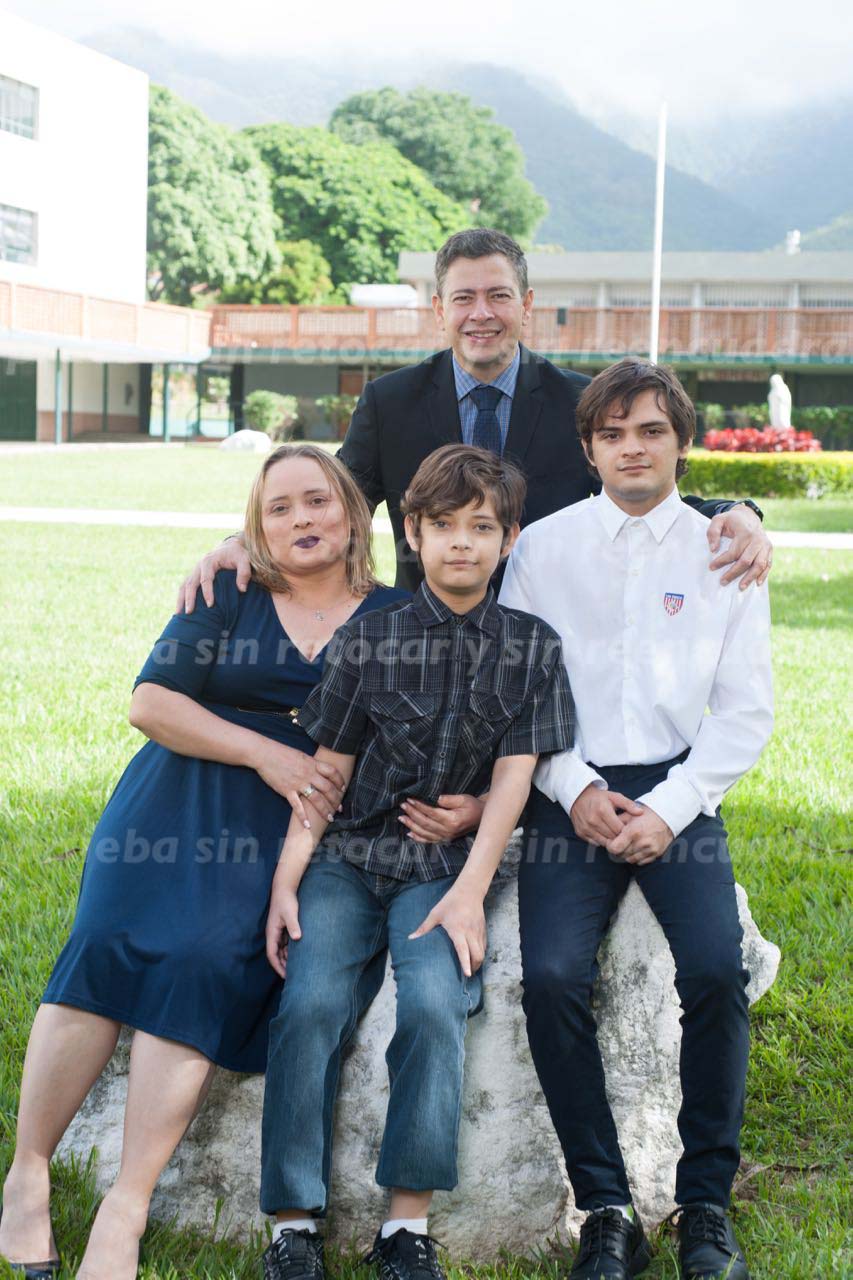The image depicts a family photo taken outdoors featuring four individuals in a scenic setting. The back row has a young man standing with short brown hair, dressed in a dark suit, blue shirt, and blue tie, smiling with his arms around the group seated in front. This group includes a woman on the left with short, flat blonde hair and a square face, dressed in a dark blue dress. She has her arm around a young boy beside her, who has curly brown hair and is wearing a dark shirt and blue jeans. Next to him is an older boy with brown hair and a square face, dressed in a white long-sleeved collared shirt and dark blue pants. All three are seated on a large white boulder with a green grassy field beneath them. The background reveals mountains, buildings, trees, and a patch of red flowers alongside a white statue to the upper right, all under a very bright sky.